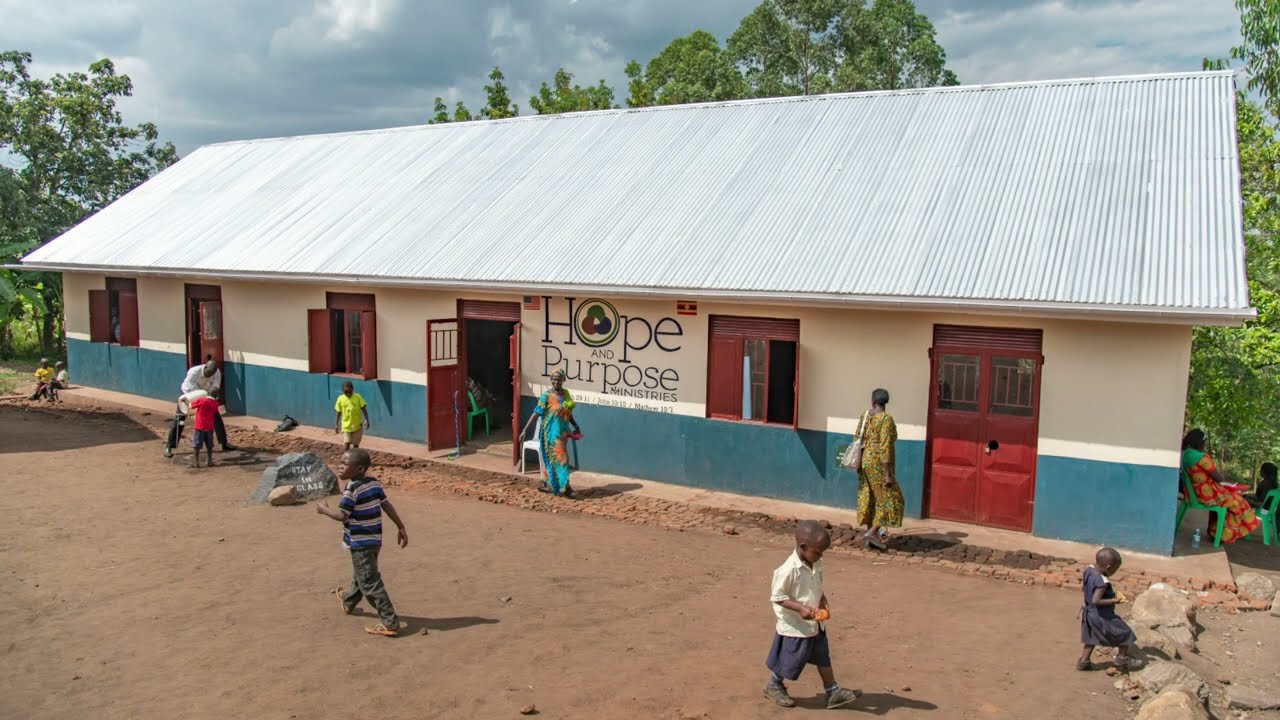In the bright outdoor image set in what appears to be a desert region, possibly Africa, a newly-built, long and narrow building is prominently featured, likely serving as a ministry or school. The building, labeled "Hope and Purpose Ministries," showcases a striped gray-silver metal roof and a stucco exterior. The upper half of the building is painted a pale peach or white color, while the lower half features a teal blue stripe. The building façade includes three red doors and three sets of red windows. The logo in the center incorporates an element inside the 'O' of "Hope," resembling hands forming a triangle or three circles. 

In front of this brightly colored structure, a group of young African children, donning various clothes including shorts and dresses, are seen walking and playing on a sandy, dirt surface. Among them is a little boy in a striped shirt. Three adults stand closer to the building, while on the right-hand side, an adult and child sit in green chairs. The scene also features a painted rock on the left-hand side with a boy in yellow behind it, standing beside another child and a man. The distant background of the image reveals green trees under a partly cloudy sky.